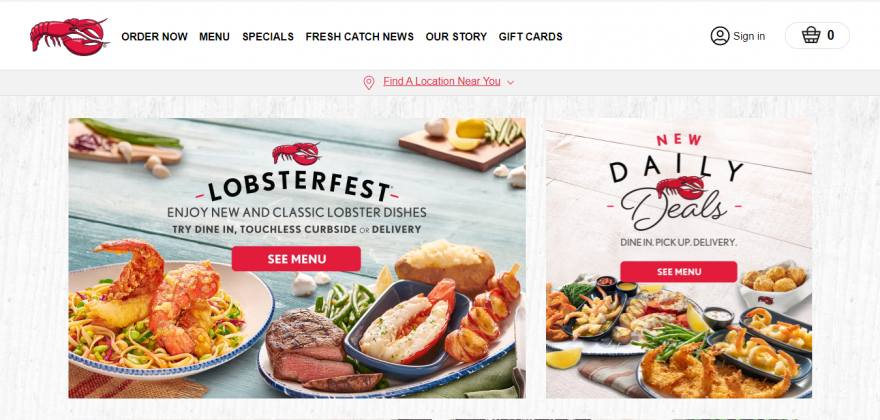The top portion of the image features a faint gray border. On the left, there is a cartoon lobster facing right. Adjacent to the lobster is a menu with black, bold, small capital letters displaying the options: Order Now, Menu, Specials, Fresh Catch, News, Our Story, and Gift Cards. On the right side of the menu is a gray circle containing a silhouette of a user icon, with "Sign In" written in gray text next to it. To the far right, there's an oval featuring a light gray border and a shopping bag icon, with "0" displayed in bold dark gray letters.

Below this is a light gray strip, centered with a red map pin icon and red text that reads "Find a Location Near You" accompanied by a dropdown arrow, all underlined in red. 

Further down, a curved banner proclaims "Lobster Fest" with a red lobster icon at the top center and red dashes on either side of the text. Underneath, in black capital letters, is the slogan "Enjoy New and Classic Lobster Dishes," followed by smaller yet bolder black text promoting "Try Dine-In, Touchless Curbside" and in non-bold script, the word "or" leading back to bold text stating "Delivery."

A red rectangular button with rounded edges in the center reads "See Menu" in bold white lettering. 

The background imagery features an array of food: to the left, fried shrimp or lobster; to the right, a steak and lobster dish. In the upper right background, there are lemons, green beans, and garlic, while the left side includes green vegetables, garlic cloves, and red onion.